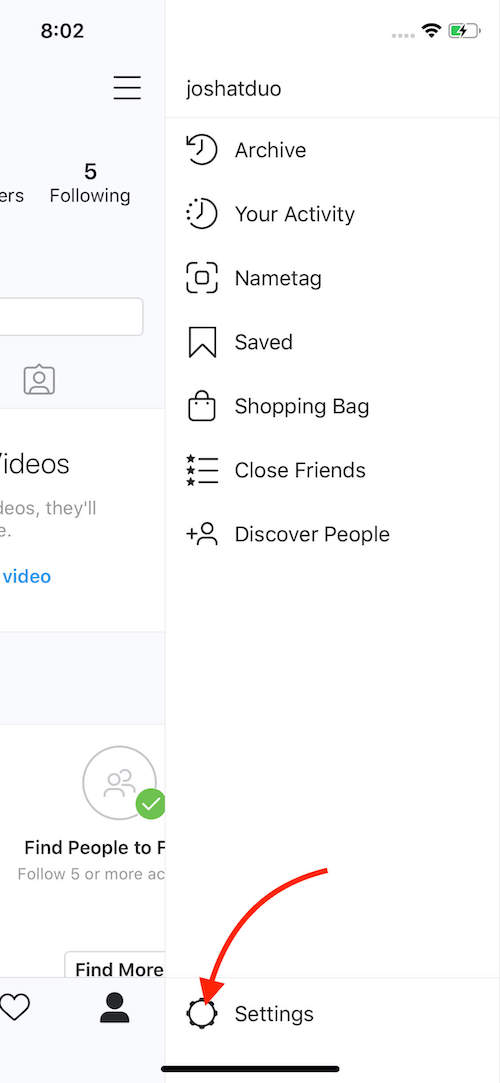This screenshot depicts the open menu interface of a mobile phone. The status bar at the top of the screen indicates the time as 8:02 AM. In the top-right corner, the phone displays a full Wi-Fi signal and a half-full battery icon with a thunderbolt, signifying that the device is currently charging. 

Positioned below the status bar, the menu is set against a clean white background with black text and icons delineating each option. The first line features the user's name, "Josh at Duo", prominently displayed. The menu options are listed as follows:

1. **Archive** - Represented by an icon of a clock, this option allows access to archived items.
   
2. **Your Activity** - This is indicated by an icon of a clock with dashes around it, summarizing your recent activities.
   
3. **Name Tag** - Accompanied by an icon of a square, for personalized tagging purposes.
   
4. **Saved** - Identified by a bookmark icon, this holds a collection of saved items.
   
5. **Shopping Bag** - Represented by a shopping bag icon, likely leading to a shopping feature.
   
6. **Close Friends** - Marked by an icon of a list with stars, for managing a close friends list.
   
7. **Discover People** - Illustrated by a human figure icon with a plus sign, for finding new contacts.

At the very bottom of the screen, there is a red arrow pointing towards the settings button, guiding the user towards further configurations and adjustments within the app.